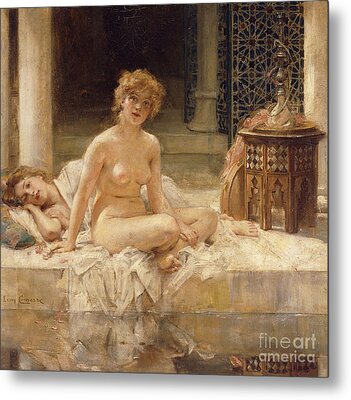The painting appears to be in the Renaissance style, depicting two white women on a white sheet in a classical setting. The woman at the center of the composition sits Indian-style, completely nude, with curly, light auburn hair. She gazes off into the distance. Beside her is an octagonal or hexagonal wooden side table adorned with intricate carvings, atop which rests a hookah. Behind her, another woman reclines with her head to the left, partially draped in the white sheet, revealing her bare arm. This second woman has slightly darker auburn hair. The background features two marble pillars and a dark blue stained glass window that transitions to lighter blue shades. In front of the window is a hookah placed on a tabletop. The painting itself has a square shape and lies on a white background. The bottom right corner bears a watermark in grayish text that reads "Fine Art America" on two lines.